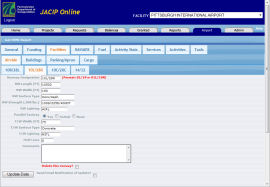The image is a screenshot of a web page characterized by an outdated design, reminiscent of early internet user interfaces, akin to old chat room communities. The page is heavily detailed, albeit with a small font size that makes the content difficult to read. 

The page title "JACP Online" is prominently displayed at the top left corner, accompanied by a green logo, likely representing the site. Adjacent to the title is a vast search bar occupying the top right section of the page. 

Directly beneath the title, there's a navigation menu with eight folder-like tabs, one of which is highlighted. These menu items oversee three rows of approximately 15 filter buttons each, with several of these buttons selected in red, indicating active filters.

The main body of the page comprises multiple rows of information fields, bearing a resemblance to an outdated Google form or an archaic data entry system for inventory like grocery store software. Each row seemingly prompts for detailed entries, such as product names, prices, and additional metadata. The overall aesthetic underscores the antiquated nature of the user interface, loaded with extensive data input options and an overwhelming amount of submenus and filters.